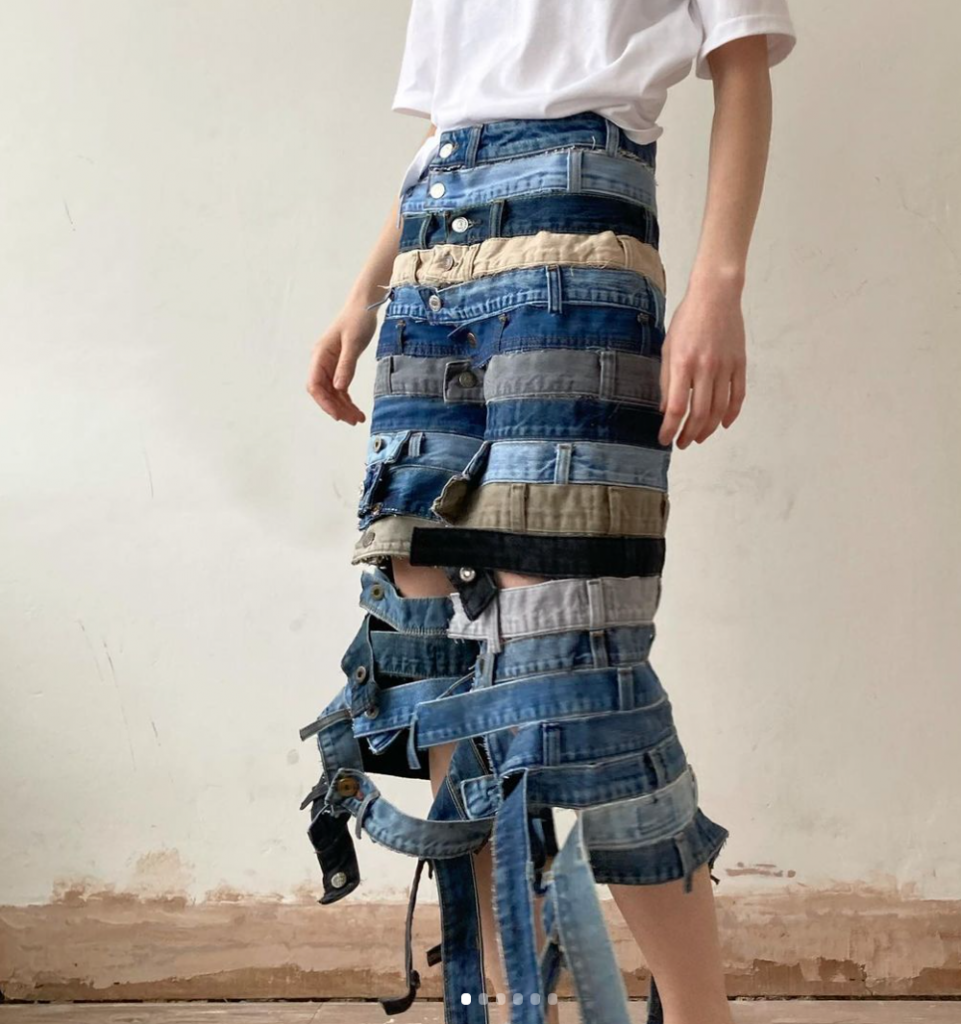The photograph captures a slim individual, likely female, from the waist down to the ankles, highlighting a unique fashion piece. The subject is wearing a tucked-in white cotton t-shirt, and the focal point is an inventive skirt made entirely from the waistbands of various pairs of jeans. The skirt consists of 18 horizontally-sewn waistbands, each representing a different color and wash, including dark blue, light blue, beige, gray, and stonewashed denim. As the waistbands descend towards the knees, they become progressively unfastened, creating a fluttering, deconstructed effect with pieces of material hanging down towards the ground. The background of the image is a muted beige tone with a subtle brown trim at the bottom, suggesting emphasis on the clothing being showcased.